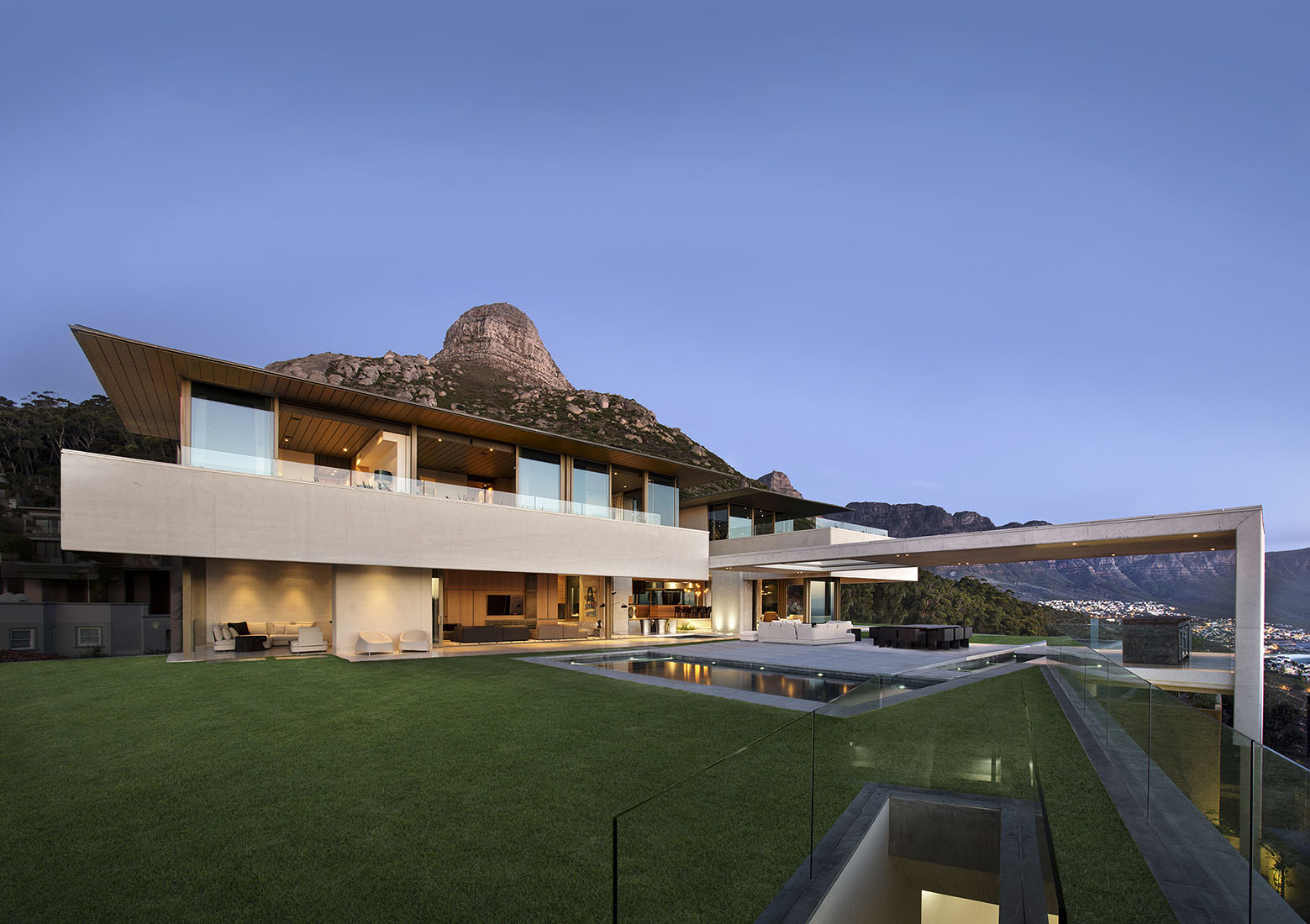The image captures a stunning, high-value mansion during a clear sunset, likely situated in California. Dominating the foreground is the sleek, ultra-modern mansion made predominantly of concrete and glass. The building is two stories high with an open-concept design, featuring luxurious white and black furniture visible through large windows. The mansion's boxy, futuristic architecture includes both a spacious lawn adorned with artificial grass and an elegant swimming pool with an adjacent jacuzzi.

Surrounding the mansion, the setting is semi-rural with panoramic views. On the left, a prominent mountain peak rises against an absolutely cloudless, deep blue sky, while additional mountain ranges stretch across the horizon to the right. A stone cliff punctuates the hillside in the middle distance, with cityscape elements faintly visible below, suggesting the house is perched on an elevated site. The comprehensive view, luxurious facilities, and meticulous landscaping created an overall impression of opulence and tranquility.